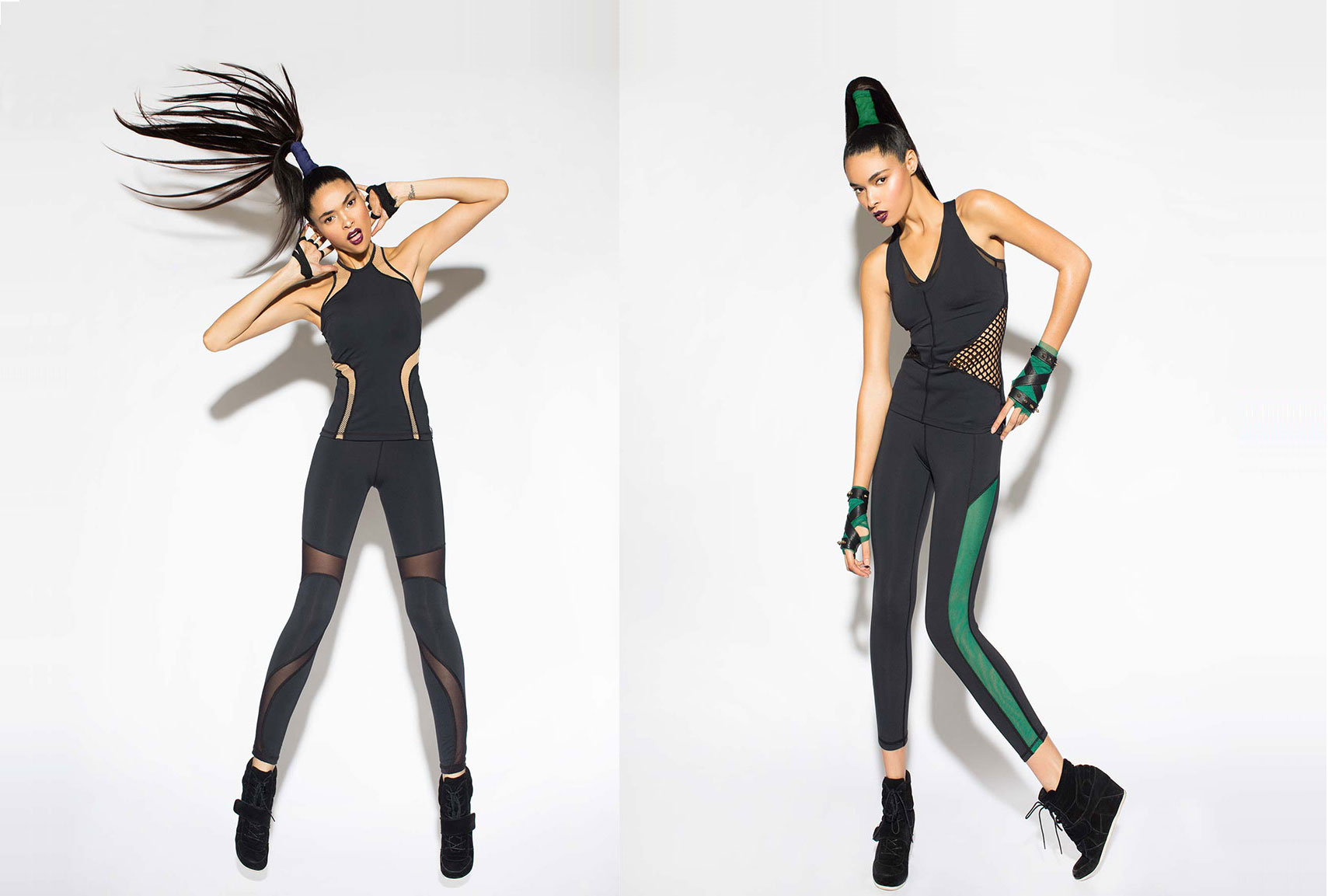This photograph features a tall, slim model striking different poses against a white background during a photo shoot. The image is presented in two parts, each showcasing a unique outfit and hairstyle.

In the first part, the model is captured standing with her legs slightly apart and her long, dark hair dramatically splayed out, likely due to the influence of a fan. Her head is tipped to the side with her hands behind her head. She is wearing a sleek black bodysuit with intricate sheer areas around the waist, thighs, and legs. The bodysuit features an elegant halter neckline with tan patterns curving from the hip towards the back, enhancing the design. Her right hand rests at her side, while her left hand is positioned on her hip. She completes this look with black boots, and her ponytail is wrapped with a blue scrunchie, accentuating the dynamic flow of her hair.

In the second part, the model is bending over her right side with her left leg bent inward at the knee. This time, she wears a black jumpsuit featuring a prominent bright green stripe running down each side of the leg. The jumpsuit is designed with a v-neckline that extends down to her belly button, with the top resembling a tank style integrated into the one-piece. Black netting forms a triangular shape from under her arms to her hips, adding a striking detail to the ensemble. The outfit is accessorized with matching black and green wristbands, and black platform shoes that give it a sporty edge. Her long ponytail, now neatly falling down her back, is tied with a green scrunchie, complementing the green accents on her jumpsuit.

Both parts of the photograph highlight the model's poised presence and sense of style, emphasizing her distinct looks with precise detailing on her outfits and coordinated accessories.